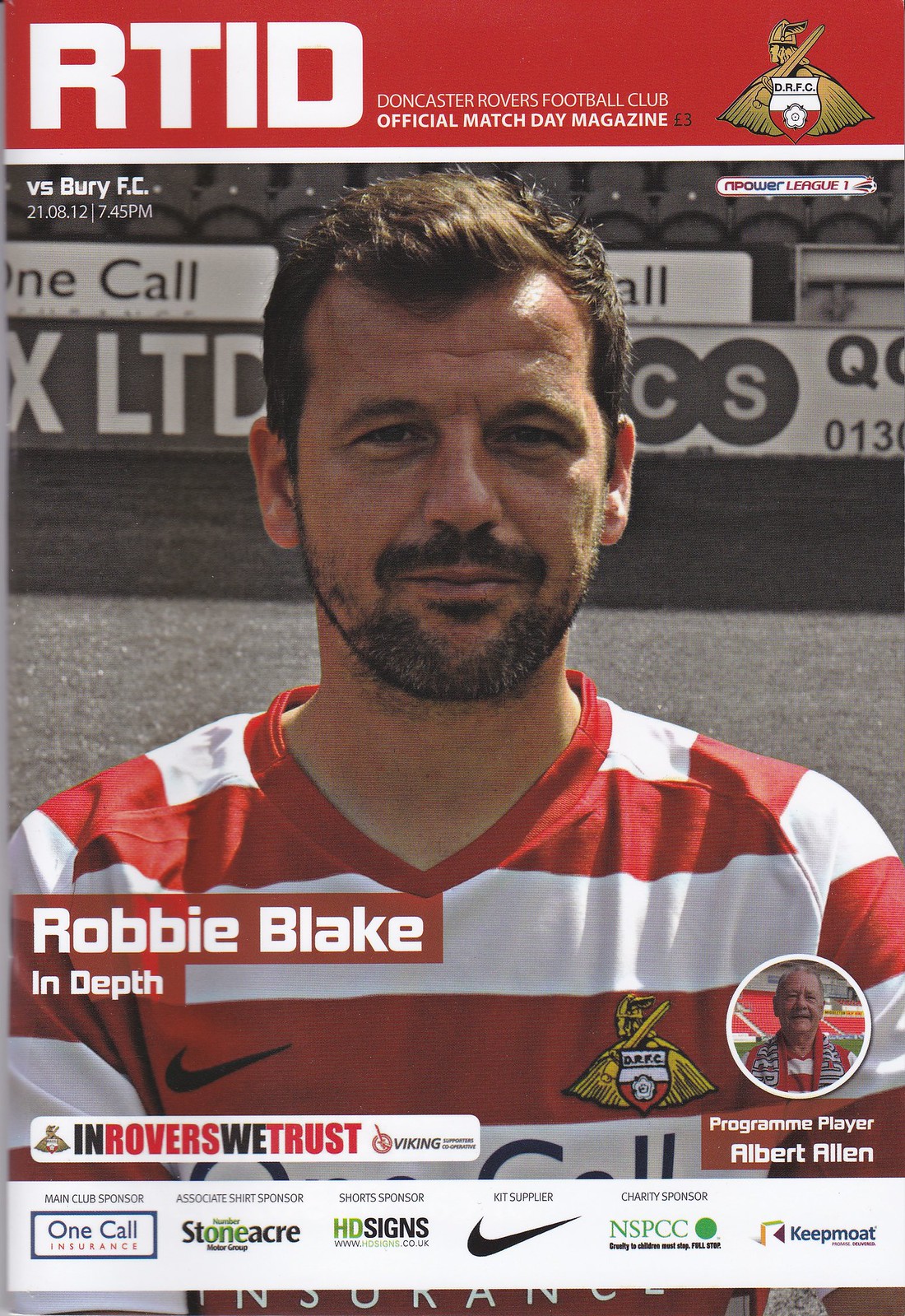This magazine cover is the official match day program for Doncaster Rovers Football Club, priced at three euros. At the top, there's a distinctive red rectangle with white text on the left reading "RT ID," and smaller text to the right stating "Doncaster Rovers Football Club Official Match Day Magazine." Alongside this text, there is an insignia of a Viking holding a sword and a DRFC shield. The main feature of the cover is a large, centered photograph of a soccer player with short brown hair and a neatly trimmed short beard, wearing a red and white striped jersey. The jersey features a Nike logo on the left shoulder and the Viking insignia on the right. Below the player's image, the text reads "Robbie Blake In-Depth: In Rovers We Trust." At the bottom of the cover, a white stripe lists various sponsors, including Nike, HD Signs, One Call Insurance, Stoneacre Motor Group, and NSPCC with the slogan "Cruelty to Children Must Stop." The jersey includes concise sponsorship credits and the logo URLs, enhancing the program's detailed presentation.